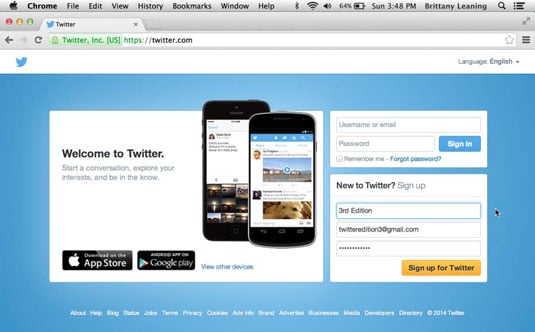This image is a detailed screenshot taken from a web browser on an Apple device, as indicated by the small apple symbol located in the top left-hand corner. Directly below the apple symbol, there are three horizontally aligned circles colored red, yellow, and green, representing the standard window control buttons (close, minimize, and maximize) on Mac devices.

The browser's single open tab is labeled "Twitter," and the corresponding URL, https://twitter.com, is visible just below the tab. The main content area of the page is centered around the prominent caption, "Welcome to Twitter." To the right of the caption are two images of cell phones displaying the website. Below the caption, on the left side, are two clickable buttons: one for downloading the app from the Apple App Store, and the other for Google Play.

On the right side of this page, there are fields available for users to log in and enter a password, along with an option to sign up for Twitter. The background of the site is light blue in color.

At the bottom right-hand corner of the page, there is a small text indicating the year 2014.

The top edge of the browser window includes standard indicators for a mobile device: the current date (Sunday), the time (3:48 PM), a battery status showing 64% charge remaining, and active Bluetooth and Wi-Fi symbols.